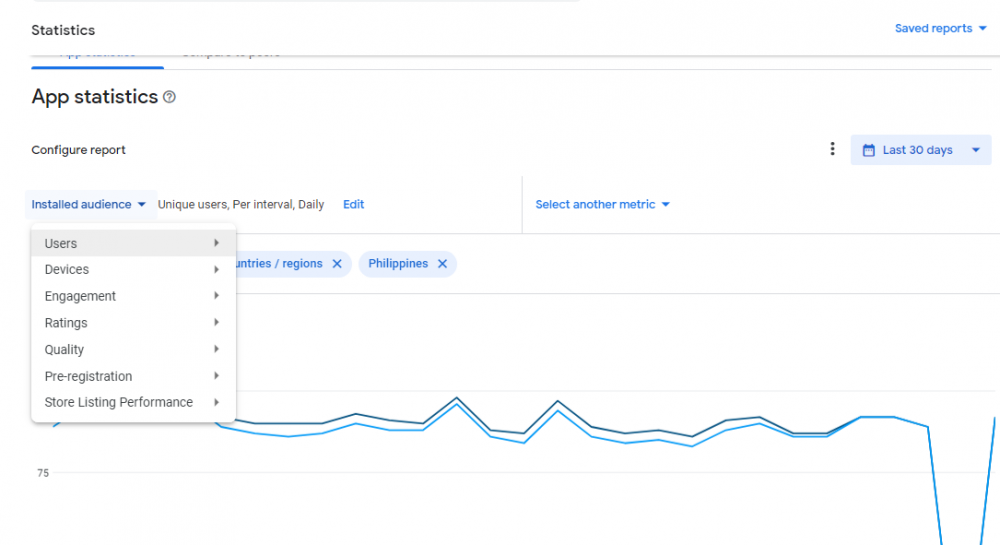This screenshot depicts a section of a developer panel, specifically the statistics page for an app. The background is white, highlighting the content. "Statistics" is prominently displayed in bold black font on the left, with "App Statistics" in slightly larger black font directly below it. A question mark icon is positioned to the right of "App Statistics", likely offering additional information or help.

Below this heading, on the left side, the phrase "Configure Report" appears in small gray font. To its right, a light blue drop-down box labeled "Last 30 days" allows for time frame selection.

Further down, two categories are listed on the left: "Installed Audience" and "Unique Users Per Interval Daily". "Installed Audience" is currently selected, showing a drop-down menu beneath it that includes options like Users, Devices, Management, Ratings, Quality, Pre-registration, and Store Listing Performance, with "Users" currently selected.

On the right side of the page, there is a large line graph showcasing data in blue and green hues. It seems to track user activity or app metrics over time. The two colored lines on the graph merge and take a sharp downturn towards the right edge of the graph, though the exact data is partially cropped from the image.